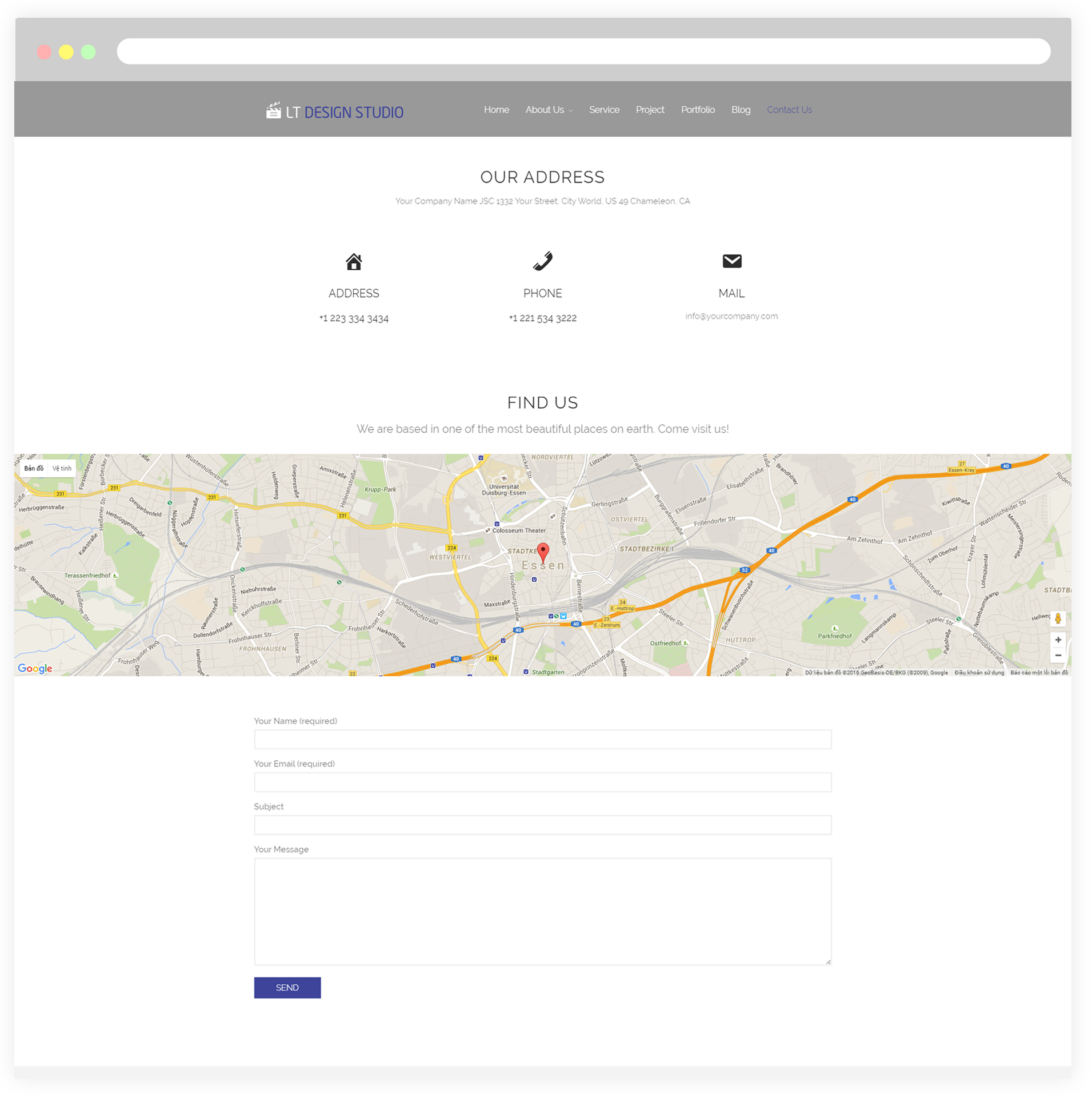The image captures a screenshot of the "LT Design Studio" website. In the upper left corner, there are three circles: the first is red, the second is yellow, and the third is green, reminiscent of window control buttons. To the right, there is an empty address bar. Beneath the address bar, a horizontal gray bar spans the top of the webpage featuring the text "LT Design Studio"—with "LT" in white and "Design Studio" in blue. To the right of this title, there are several buttons labeled "Home," "About Us," "Blog," "Contact Us," and other smaller, unreadable options.

The main content area has a white background. At the top center, the heading "Our Address" is prominently displayed, followed by some descriptive text. Below this heading, specific contact details are listed: 

- An address with a "home" icon above it
- A phone number accompanied by a "phone" icon
- An email address represented by an "envelope" icon

Additionally, there is a section labeled "Find Us," featuring a location map. At the bottom, there is a box to input information and send a message.